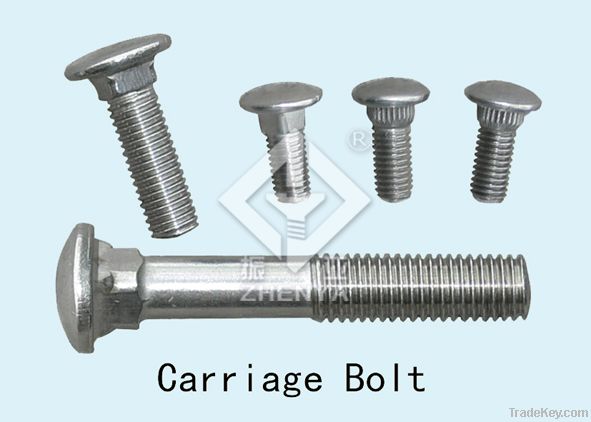The image features five metal bolts of varying sizes against a very light pastel blue or green background. At the bottom of the image, in bold black sans serif font, the text reads "Carriage Bolt." The bottom right corner displays a light gray URL: tradekey.com. Dominating the center of the composition, a large bolt lies horizontally with its head on the left and threaded end on the right. Above this bolt are four additional bolts positioned vertically, heads facing upward. The farthest left bolt is the largest, slightly tilted, while the remaining three are of the same size. A watermark in the middle of the image showcases a diamond-shaped symbol with a screw inside, accompanied by Chinese or Japanese characters and the word "Zenya" in English. To the right of this watermark is a circle containing an "R," indicating rights reserved.